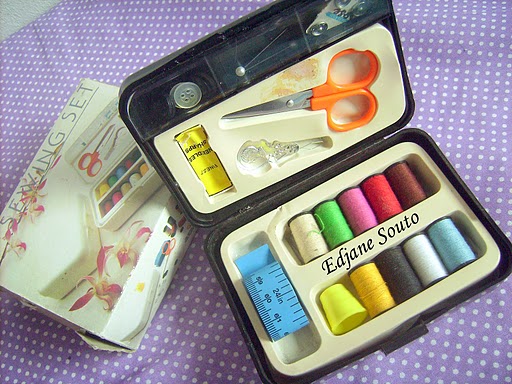This color photograph, taken in landscape orientation, showcases an open sewing kit angled in the bottom right corner of the frame. The sewing kit features various colored threads, including off-white, light green, pink, rose, brown, blue, white, gray, and yellow, arranged in two rows of five spools each with the words "Edging Saute" in black text between them. A yellow thimble, a light blue measuring tape, and assorted buttons and pins occupy other compartments within the kit. The lid of the kit, embedded with orange-handled scissors, extends toward the top of the image, which is cropped at the corner. A box labeled "Sewing Set" in all caps and featuring a photograph of the sewing kit is positioned behind and to the left of the kit, also at an angle. Both items rest on a background composed of a light purple cloth adorned with rows of white dots, emphasizing the realism and detailed style of product photography used in this image.